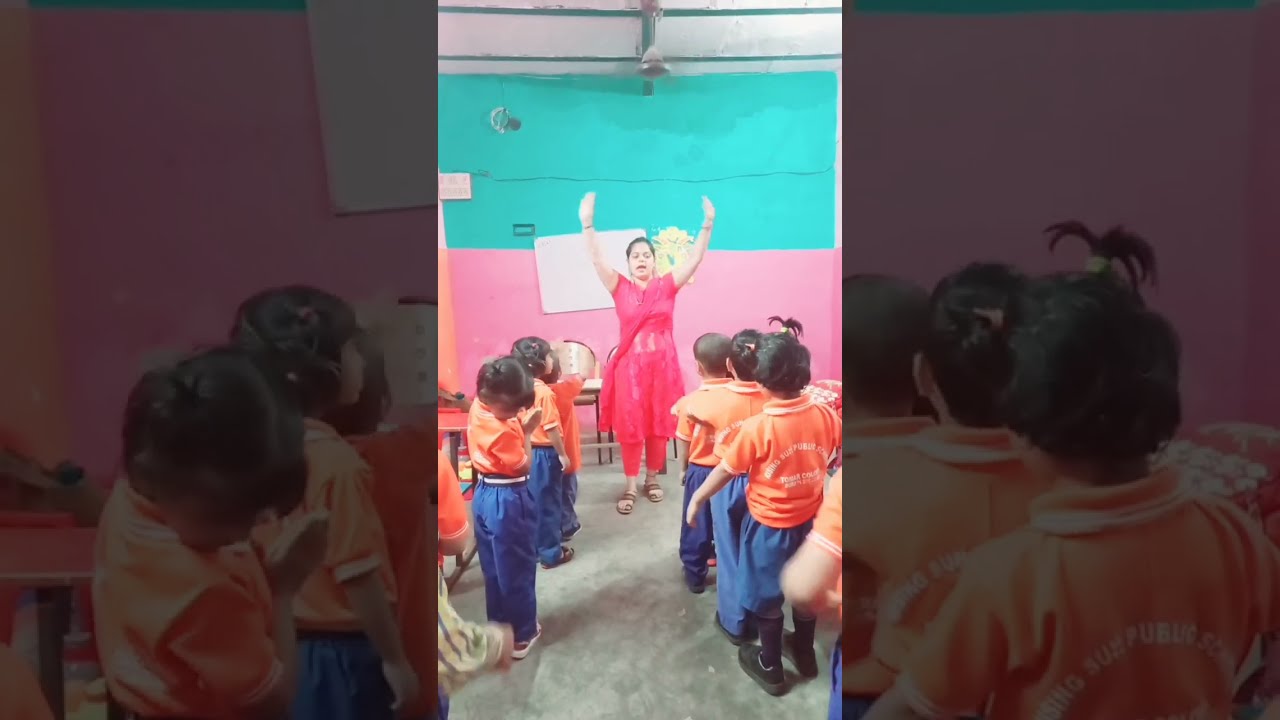The image features a vibrant, well-lit classroom divided into three parts. Dominating the center is a clear and bright scene: a woman who appears to be a teacher stands confidently with her arms raised in what seems to be a gesture of instruction or exercise demonstration. She is dressed in a red outfit that resembles a sari paired with long pants, and she wears sandals. Flanking her are children on both sides, organized into straight lines; they are dressed in matching orange shirts and blue pants, indicative of a school uniform. Each child has dark hair, many styled in small ponytails, and they watch the teacher intently, suggesting she is leading them in an activity.

The background showcases a classroom setting with a dual-colored wall— the top half painted aqua and the bottom half pink. Behind the teacher, a green and red flag is partially visible, along with what seems to be a whiteboard. This middle section stands out in brightness and clarity.

On the left and right sides of the image, shadows create a darker, almost blurred effect, echoing a zoomed-in, higher-intensity version of the central scene, making the children appear larger and less focused. The image gives an impression of energy, discipline, and a vibrant school atmosphere.